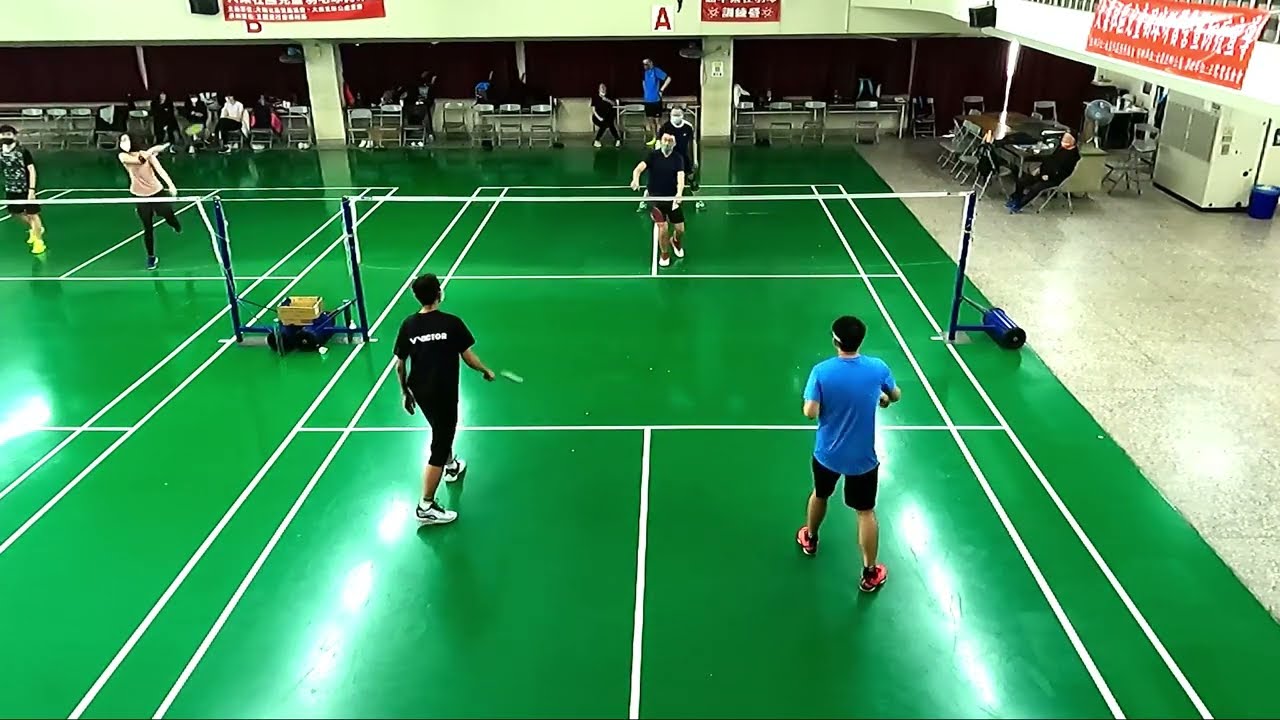This is an indoor pickleball court with vibrant, emerald green painted cement floors and white lines. The main focus is on a court where four male players, wearing black t-shirts and shorts, are actively engaged in a game. One player stands out in a blue t-shirt. They are positioned across a small net, and all are holding small rackets distinctive to pickleball. Adjacent to this main court, another court is visible, showing a woman swinging her racket next to a man, suggesting they are part of a mixed-gender team. The indoor venue is well-lit with overhead lighting that reflects off the floor, enhancing visibility. Background features include red banners on the sidewalls, columns, and a row of fold-out chairs. Among the chairs, a few people are seated while one person remains standing, adding to the lively atmosphere of the setting.